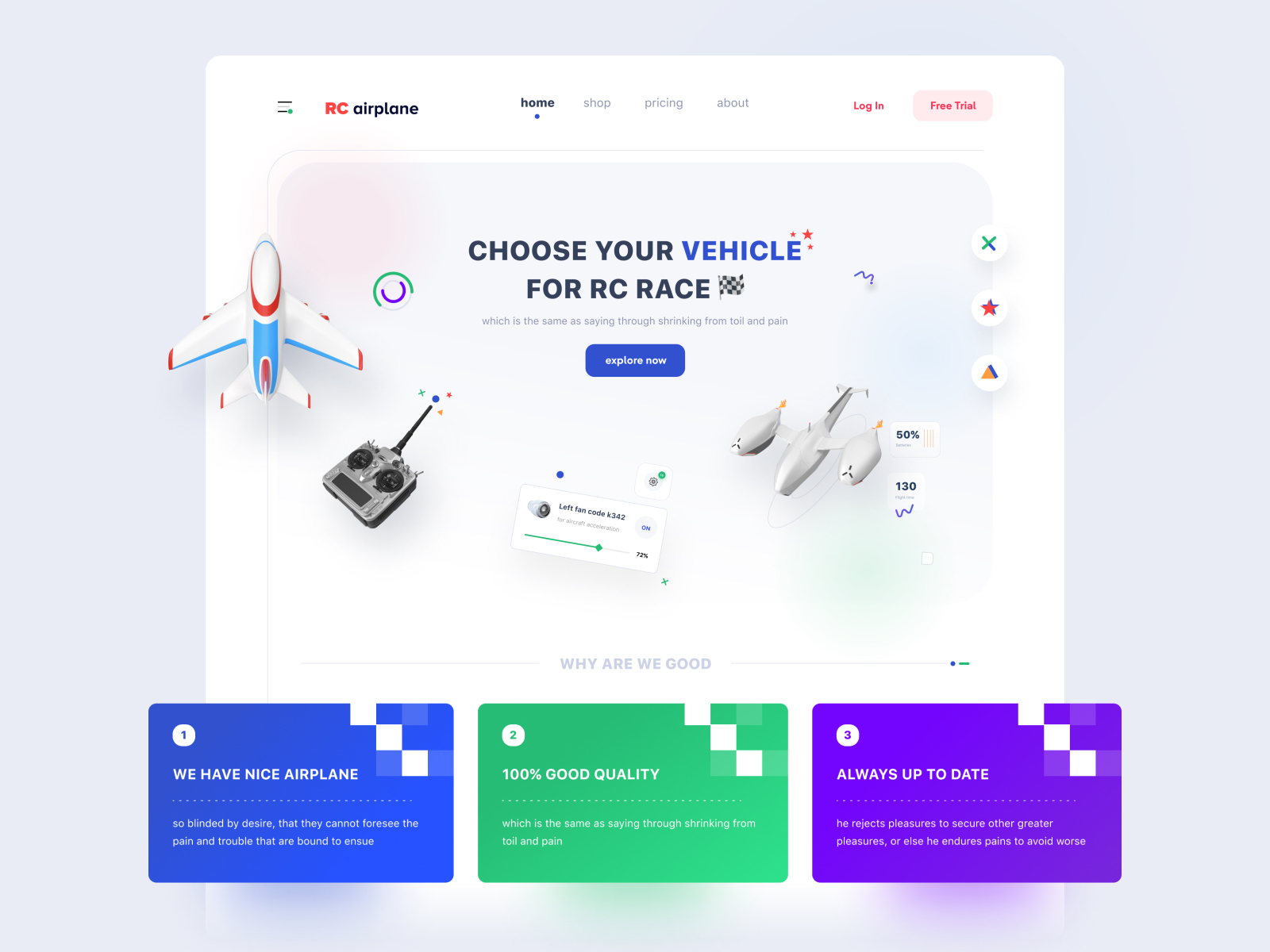The screen capture features a website titled "RC Airplane." Dominating the center of the screen is a bold prompt urging users to "Choose Your Vehicle for RC Race," accompanied by a checkered flag graphic symbolizing competition. Below this message, there is a small blue button, the text on which is indistinct due to its size. Displayed prominently are various images of model airplanes, each equipped with remote controls, designed for outdoor flying activities such as in a park.

The website also showcases a tagline that boasts, "We have nice airplanes, 100% good quality, always up-to-date." Additionally, it poses the rhetorical question, "Why are we good?" This is presumably meant to highlight their commitment to quality and customer satisfaction. The page suggests that users can click on the displayed items to learn more or make a purchase. The overall content and visuals indicate that the website sells a variety of RC (remote control) vehicles, including drones, race cars, and airplanes, making it a recommended destination for enthusiasts looking to buy such toys.